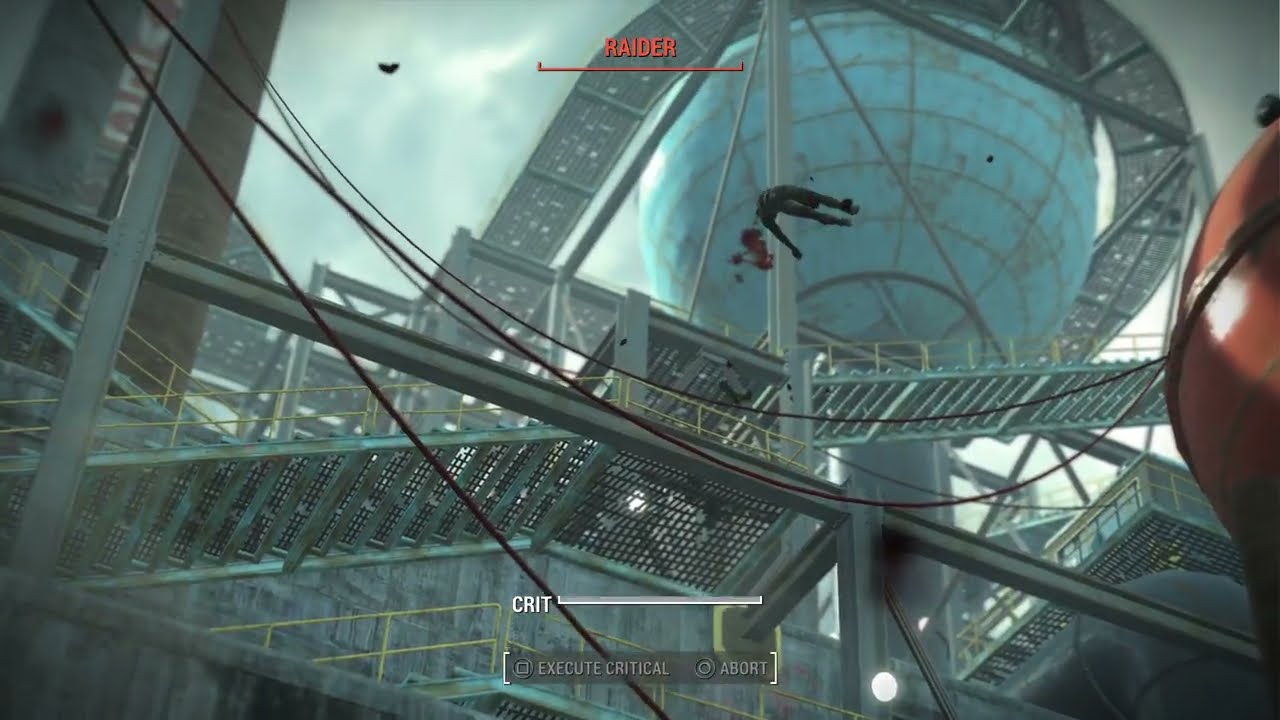The image is a detailed screenshot from a video game, showcasing an outdoor metallic structure that resembles a complex assembly of stairways, pathways, and catwalks, reminiscent of a roller coaster, with looping tracks and poles. The towering building is predominantly blue and grey, with a large blue circular bowl at the top, accompanied by ropes and another smaller red bowl visible at the right corner. A character dressed in black appears to be flying or being flung across the screen, their limbs sprawled outwards. The building seems to be set against a dark, possibly night sky. Prominently, at the top-middle of the screen, the word "Raider" is displayed in red text, while the bottom-middle features a grey bar with the commands "Crit," "Execute Critical," and "Abort" inscribed on it.